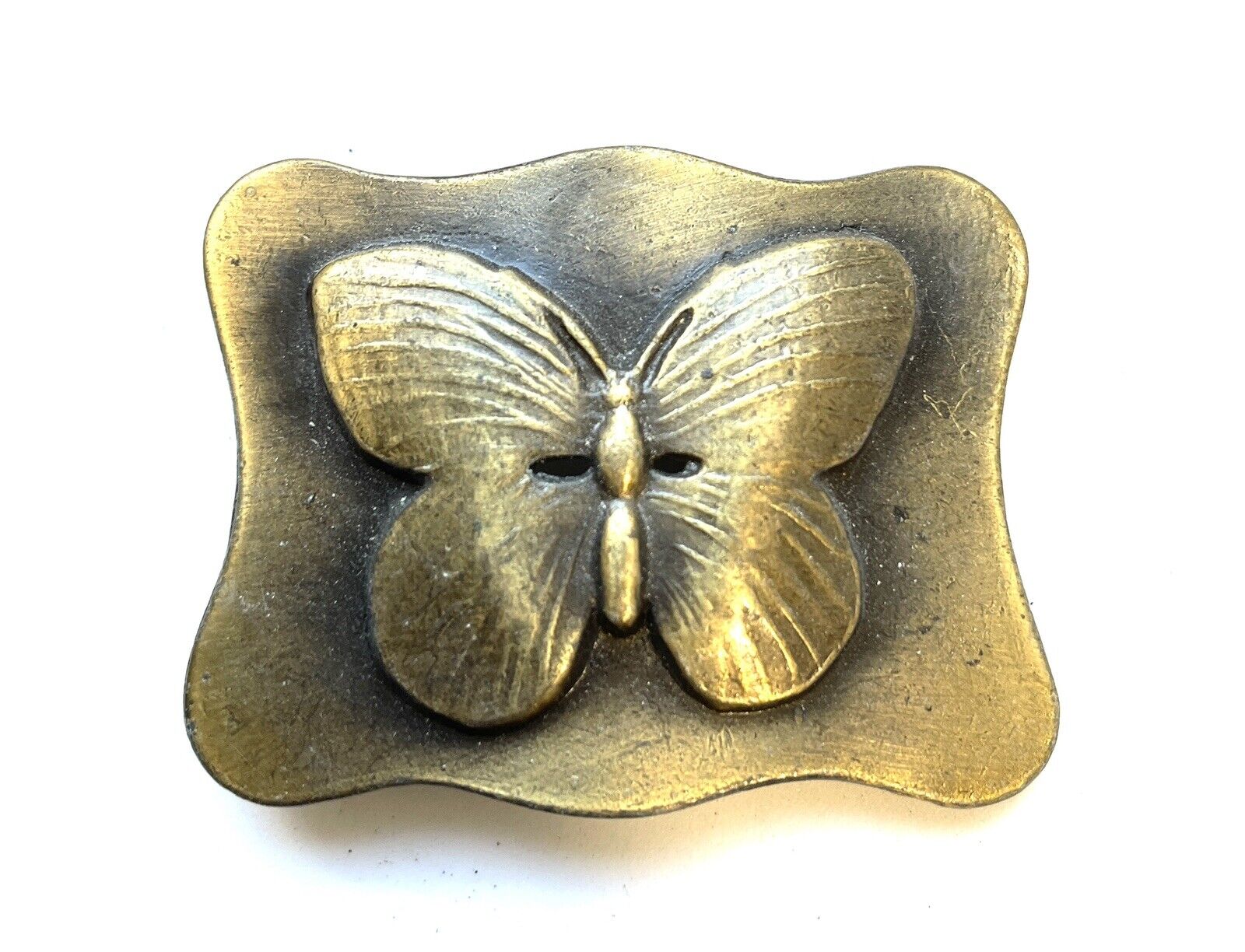The image depicts a gold-plated, wavy rectangle-shaped piece of metal with black and gold coloration. Centrally positioned on this ornate item is an intricate engraving of a butterfly with veiny wings and antennae. The butterfly's wings, which are entirely gold, nearly touch the edges of the metal piece on both sides. The metal's surface features smooth, undulating curves that add to the visual appeal of the object, suggesting it could be an exquisite piece of artwork or jewelry. Around the butterfly, the background is a stark, empty white, drawing full focus to the central design.